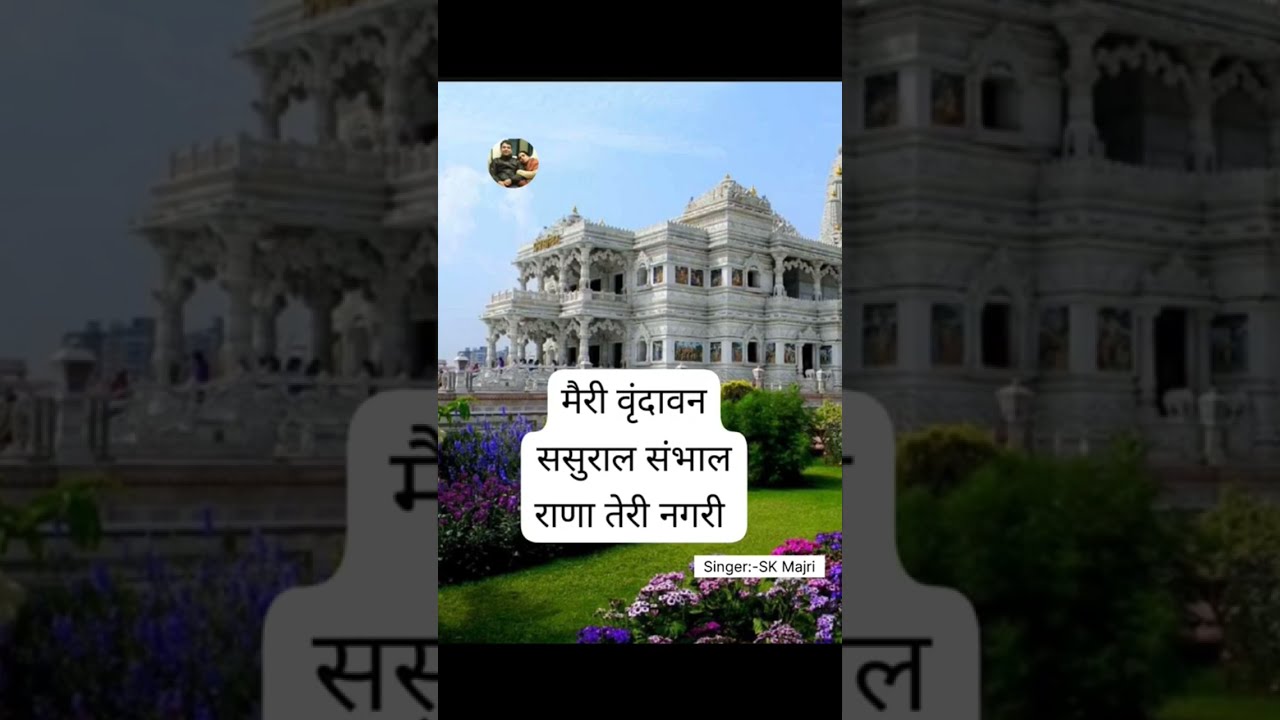The image features a grand, ornate white building reminiscent of a castle, likely located in India due to the presence of Indian Hindu writing prominently displayed in the center. The architecture is elaborate, with multiple decks, an abundance of columns and windows, and detailed stonework. The majestic building is surrounded by meticulously maintained gardens, filled with vibrant flowers in shades of purple and pink, and well-manicured green lawns. Taller flowers and shrubs add to the lushness of the scene. The background showcases a clear blue sky, enhancing the overall beauty. In the upper left corner, a small circular inset possibly depicts the photographer. At the bottom right, there is text in Indian script, suggesting this image may have been shared on social media, perhaps featuring a quote or lyrics from a popular singer.